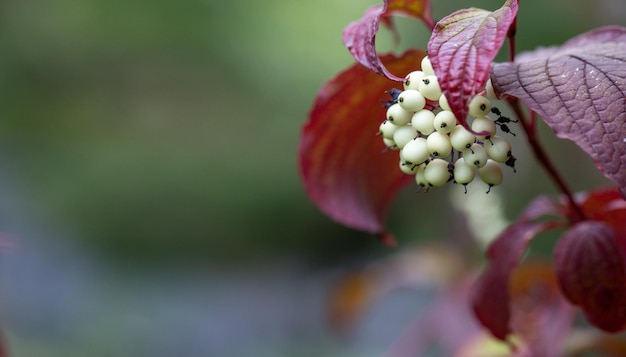This captivating close-up photograph features a wild berry plant with striking deep maroon-red, almost burgundy, leaves that curl gently at the tips. The reddish stem of the plant extends diagonally from the lower right corner to the central upper edge. The focal point of the image is a dense cluster of about 20-25 white berries, each with small black stems, emerging from the base of one of the leaves. The leaves are richly detailed with slightly darker veins that add depth and texture. The background, a mixture of green hues, suggests a lush, possibly wooded area, or garden, and is beautifully blurred to draw attention to the vivid details of the plant. The entire composition creates a striking contrast between the bold colors of the plant and the soft, diffuse greenery behind it.